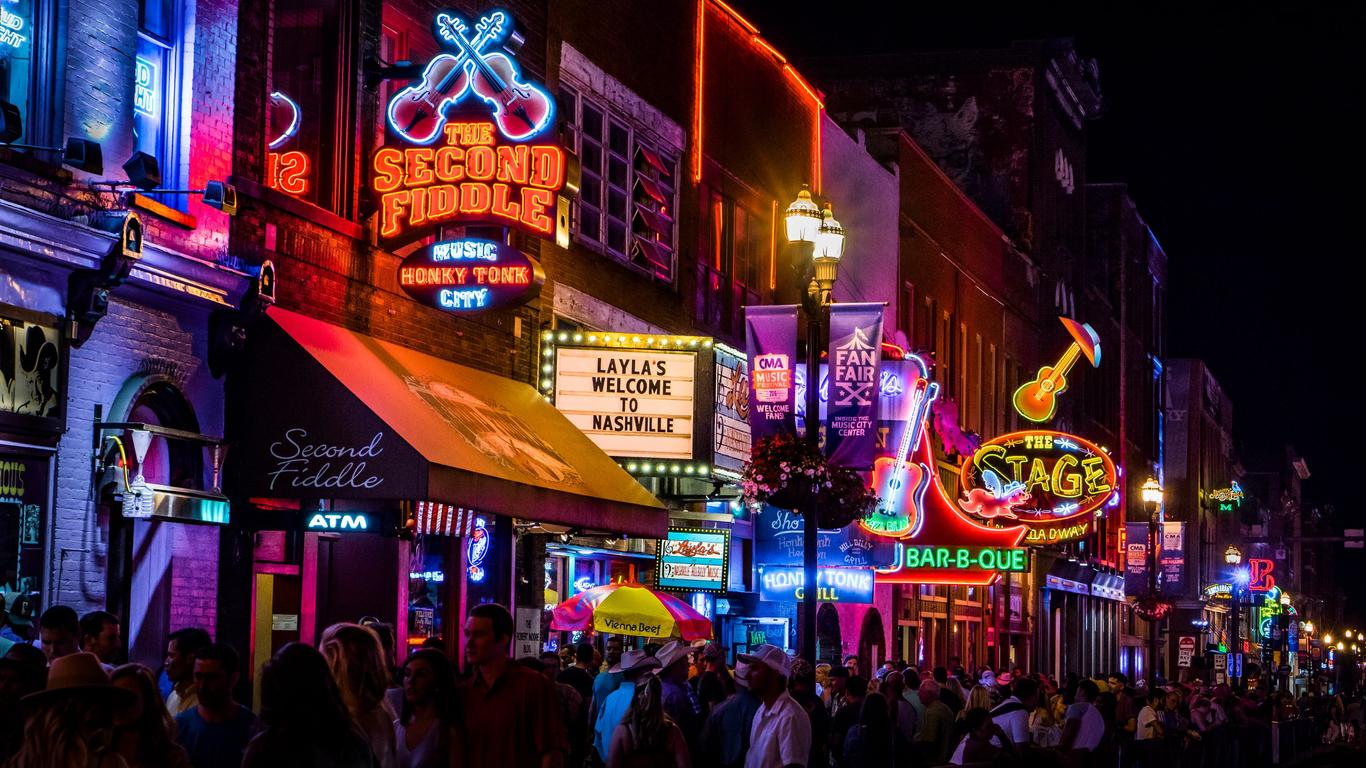This vibrant nighttime photograph captures the bustling energy of downtown Nashville, Tennessee. The scene is a veritable showcase of neon lights and busy streets, teeming with people enjoying the city's nightlife. The most prominent building features a neon sign with two crisscrossed violins and the name "The Second Fiddle Music Honky Tonk City," along with an awning below that says "Second Fiddle" and an ATM sign. Flanking this are various other brightly lit signs, including a marquee that reads "Leila's Welcome to Nashville," confirming the location. Further along, there are are numerous other establishments, each with its own colorful signage: a green neon "Barbecue" sign, a "The Stage" sign adorned with a neon guitar topped with a cowboy hat, and a banner announcing "Fanfare X." The street, bathed in the glow of these myriad lights, is filled with people who are either strolling along the sidewalk or examining the lively storefronts. The clear night sky enhances the vibrancy of the neon colors, encapsulating the spirited nightlife of Nashville.